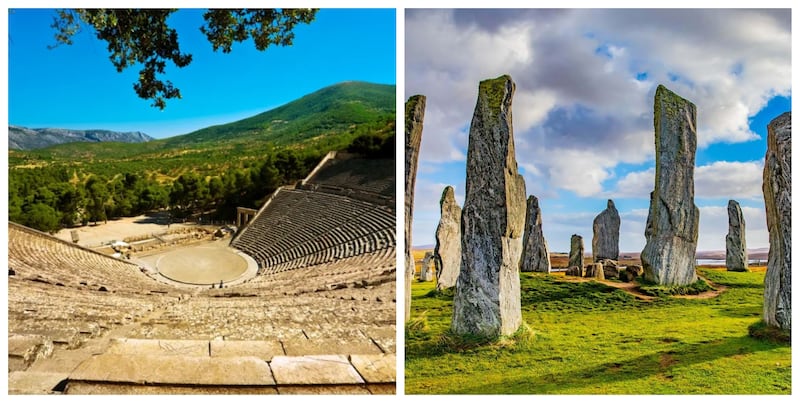The composite image comprises two photographs placed side by side, each showcasing distinct ancient landscapes under vivid blue skies. 

The photo on the left captures a worn Roman amphitheater made entirely of sandy-colored stone. The viewer's perspective is from a high vantage point beneath overhanging tree branches, looking down into the circular center stage of the amphitheater. Beyond this ancient ruin, green rolling hills, scattered trees, and distant mountains frame the scene, adding depth and a sense of historical context.

The right-hand photo portrays a grass-covered field featuring nine towering, vertical stone structures reminiscent of Stonehenge, though arranged more randomly and appearing slightly weathered with gray and white striations. The bright green grass contrasts sharply with the vivid blue sky, filled with scattered gray and white clouds. The stones cast leftward shadows, indicating the sun is positioned towards the right. In the background, harvested fields and a hint of distant water can be seen, though the expansive sky and monumental stones dominate the scene.